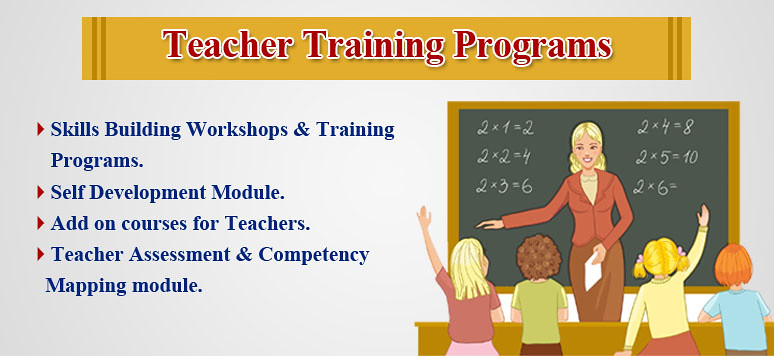The image titled "Teacher Training Programs" features a detailed layout. The heading is prominently displayed at the top against a light blue background. Below the heading, on the left side, four key points are listed: Skills Building Workshops and Training Programs, Self-Development Module, Add-on Courses for Teachers, and Teacher Assessment and Competency Mapping Module. On the right side of the image, there's an illustrated scene depicting a classroom. In the drawing, a blonde-haired teacher, dressed in a brown long-sleeve shirt and skirt, stands in front of a blackboard framed with brown wood. The blackboard displays a series of multiplication equations ranging from 2 times 1 equals 2 to 2 times 5 equals 10, with 2 times 6 partially completed. Four students are seated in the classroom, two of whom have their hands raised. The students appear to be a mix of two boys and two girls, characterized by various hair colors: the girls have blonde hair, one boy has brown hair, and the other boy has red hair. The teacher appears to be engaging the class and possibly calling on one of the students with their hand raised.